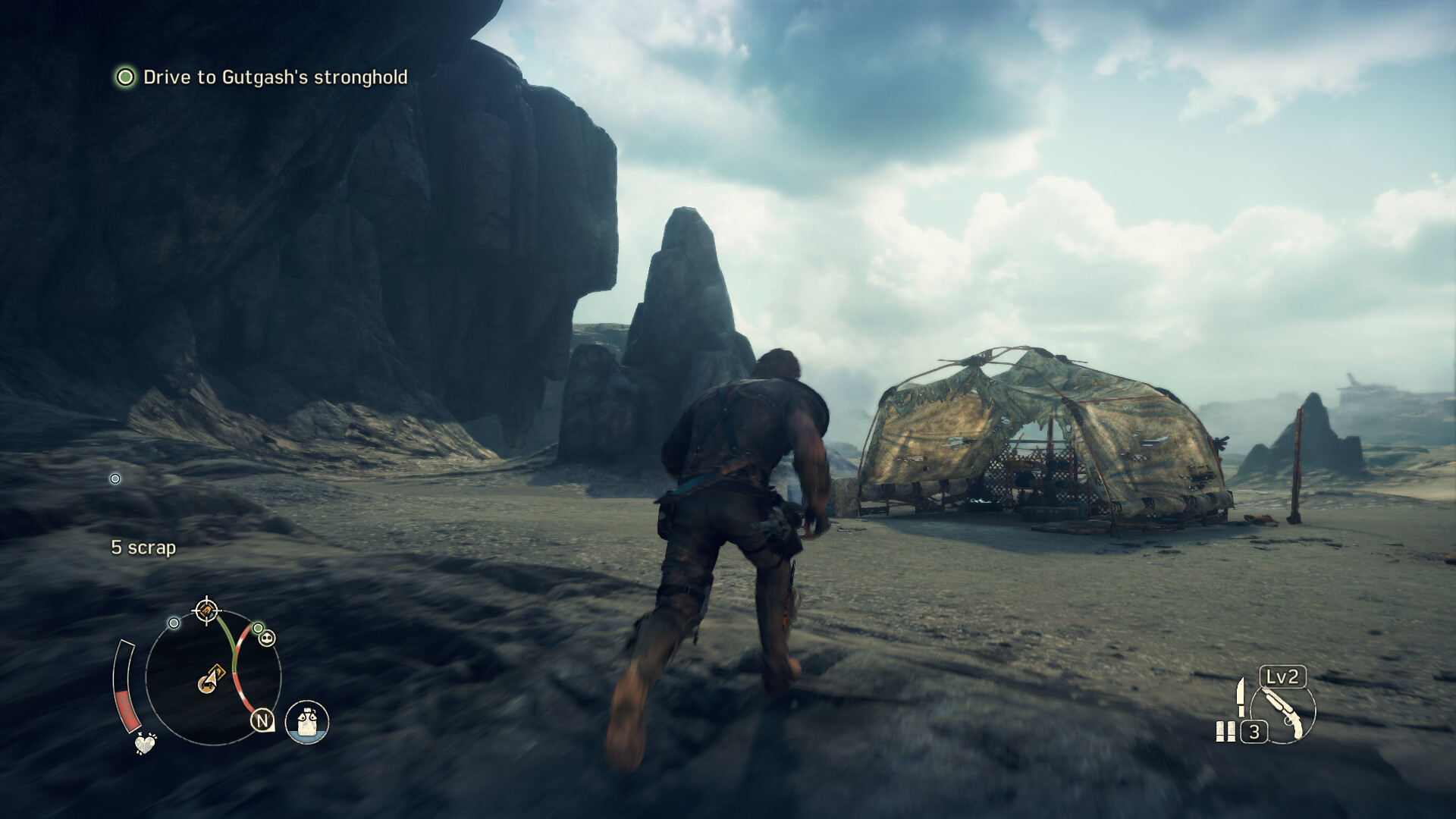This is a detailed screenshot from an unrecognized video game, possibly Mad Max. At the center and bottom half of the image, a man is running barefoot towards a tattered tent made of a hide-like material. He is wearing dark, tattered clothes that are muddy and torn, suggesting a harsh, rugged environment. The man's left foot is slightly blurred, indicating motion. He is on a textured surface mixing beige, tan, light brown, and shades of gray.

In the bottom left corner, a circular mini-map indicates pathways with red and green lines, displaying a gold triangle marking the player's position near a smaller orange square. Adjacent to it, a curved health bar, about halfway filled with red, denotes the player's vitality. Above this is a white heart symbol and five scrap icons. 

On the bottom right, a white graphical image features a level 2 shotgun, with "LV2" written above it, accompanied by a number 3, an image of a knife, and shotgun shells. The sky in the background is blue and overcast, with patches of white and dark blue clouds, hinting at an impending storm. In the top left corner, white text instructs the player to "Drive to Gut Gashes Stronghold."